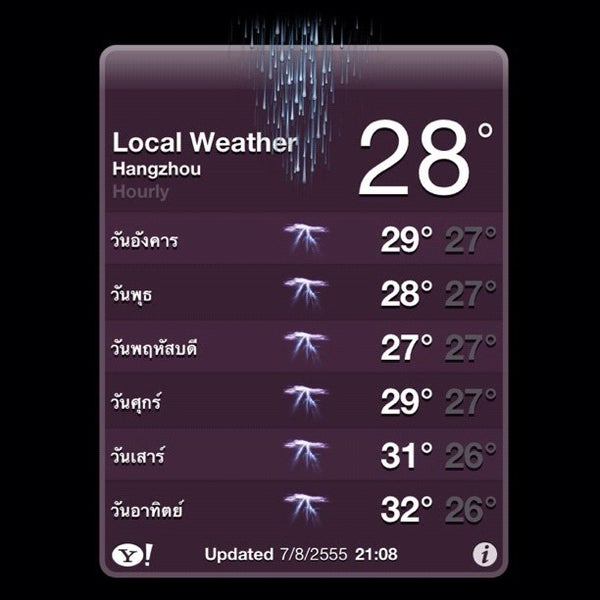A detailed image description of a weather forecast from Yahoo Weather for Hangzhou. The forecast prominently displays a temperature of 28 degrees in large font, indicating the current weather conditions. Arranged vertically on the left side of the image are the names of upcoming days written in a different language. The main image shows raindrops, signifying that it is currently raining in Hangzhou. 

On the right side, the forecast for each day includes both high and low temperatures. The icon for Yahoo can be seen in the lower-left corner of the image, while an information symbol (an 'I') is located in the lower-right corner. The update timestamp in military time is noted as 21:00:08 on 7-8-25-5-5. The background of the image is predominantly black, with a dark purple section highlighting the local weather details.